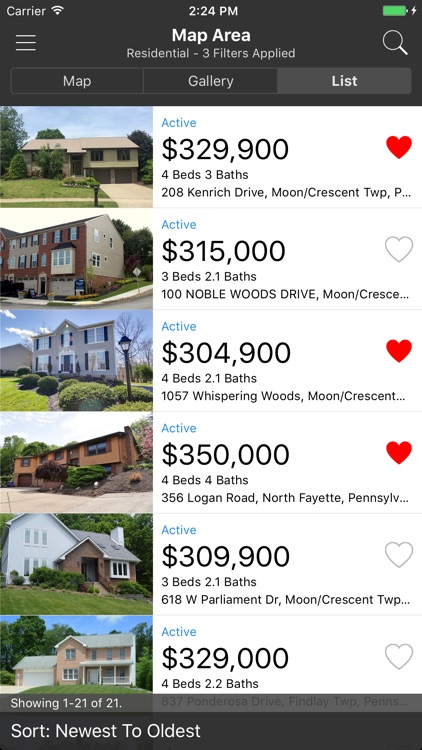Here is a detailed and cleaned-up caption for the described image:

---

The image appears to be a screenshot from a mobile phone displaying a real estate listing app at 2:24 PM, with full battery and cellular carrier indicated. At the top of the screen, there are three tabs labeled "Map," "Gallery," and "List," with the "List" tab currently selected. With three filters applied, the listings are categorized under "Residential."

1. **208 Kenridge Drive, Moon Crescent**:
   - Status: Active
   - Price: $329,900
   - Bedrooms: 4
   - Bathrooms: 3
   - Description: The house, favorited by the user, features a yellowish hue with some brick and brownish wood accents. It sits on a traditional green lawn with a clear sky in the background.

2. **100 Noble Woods Drive, Moon Crescent**:
   - Status: Active
   - Price: $315,000
   - Bedrooms: 3
   - Bathrooms: 2.1
   - Description: This unfavorited listing appears to be part of a larger complex or condominium. It features more brick and a visible garage, suggesting a modern style.

3. **1057 Whispering Woods, Moon Crescent**:
   - Status: Active
   - Price: $304,900
   - Bedrooms: 4
   - Bathrooms: 2.1
   - Description: This favorited home is bluish with large glass windows, set on a nice lawn with a lamp post and a blue sky backdrop.

4. **7356 Logan, North Fayette, Pennsylvania**:
   - Status: Active
   - Price: $350,000
   - Bedrooms: 4
   - Bathrooms: 4
   - Description: Also favorited, this home has a brown, woodish-tan exterior and appears to be situated on an embankment.

5. **618 West Parliament Drive**:
   - Status: Active
   - Price: $309,000
   - Bedrooms: 3
   - Bathrooms: Not specified
   - Description: The house features a blend of brick and light blue accents.

6. **837 Ponderosa Drive**:
   - Status: Active
   - Price: $329,000
   - Bedrooms: 4
   - Bathrooms: 2
   - Description: This home has a tannish-brick exterior, a nice lawn, and an attached garage.

---

This detailed caption provides a clear, organized summary of each property listed in the real estate app screenshot.